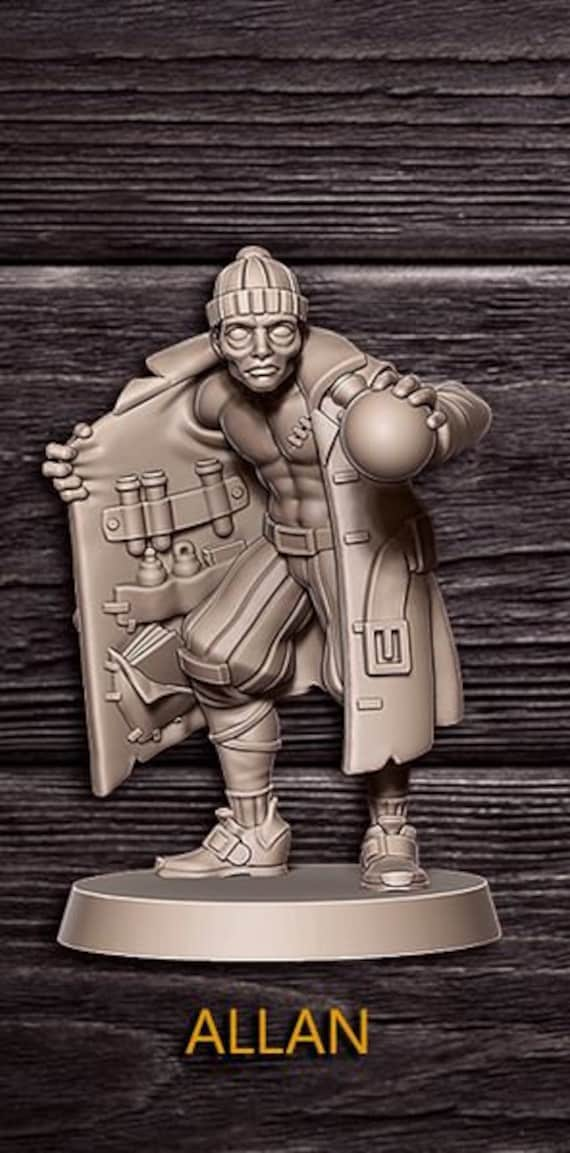The image depicts a detailed sculpture of a man, crafted from a grey or pewter-colored metal, possibly bronze. The figure is positioned against a rich, dark brown wooden surface composed of three visible planks arranged horizontally. The base of the sculpture displays the name "Allen" in yellow capital letters. The man is portrayed wearing a trench coat, pants, and sneakers with buckles. Notably, he is topless beneath the coat, revealing bandages or stitches across his chest. He dons a beanie and holds a round-bottom flask in his left hand. His right hand is pulling open the trench coat to reveal an assortment of items inside, including what appear to be test tubes near the top, grenade-like objects in the middle, and a book at the bottom.